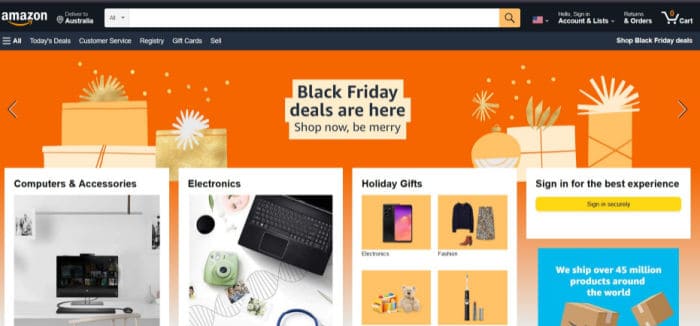The screenshot captures the Amazon.com homepage, prominently featuring their Black Friday promotion. The top third of the page is predominantly orange, with an irregularly shaped white box in the center. Inside this box, written in a bold black font, are the words "Black Friday. Deals are here, shop now, be merry." Flanking this central message are illustrations of presents, depicted in shades of gold and white, tied with blue ribbons.

Beneath this promotional banner, three distinct categories are displayed in white boxes. The first category on the left is "Computers & Accessories," accompanied by an image of a desktop computer and keyboard. In the center, the "Electronics" category showcases a laptop with a black keyboard and surface. To the right, the "Holiday Gifts" category features a white box containing four squares with a light orange background. These squares display images of a smartphone, a skirt, a boot, and a black jacket. Lastly, in the "Toys" section, there is an image of a teddy bear, and another object in the far right corner that is not clearly identifiable.